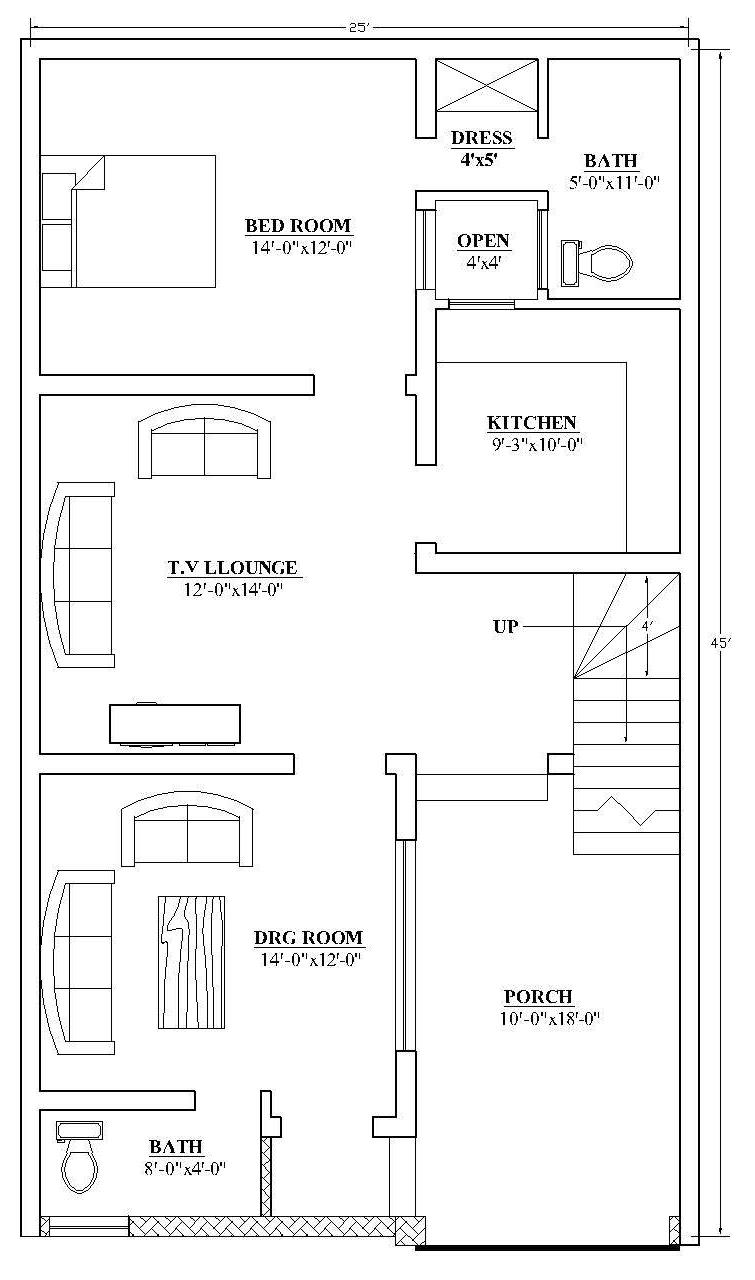This detailed floor plan illustration of a rectangular house shows a variety of clearly labeled rooms and furniture layouts. Starting from the top left, the main bedroom features a bed with two pillows, positioned in the center of a square labeled "Bedroom." Adjacent to this is a dressing area marked "Dress Table," and a bathroom illustrated with relevant icons such as a toilet.

Exiting the bedroom and moving towards the right, there's a kitchen area directly below the bathroom, depicted as a small square. Continuing right leads to the lounge area, which includes a two-seater couch at the top, a three-seater couch on the left, and a coffee table below. This area is centrally labeled "TV Lounge."

To the right of the TV lounge, there's an opening that appears to be stairs leading down to a porch, identified as "Porch."

On the left side of the porch lies another seating area labeled "DRG Room," which contains a two-seater couch at the top, a three-seater couch on the left, and a small coffee table in the center. Finally, located towards the bottom of the layout is an additional bathroom, highlighted with another toilet icon.